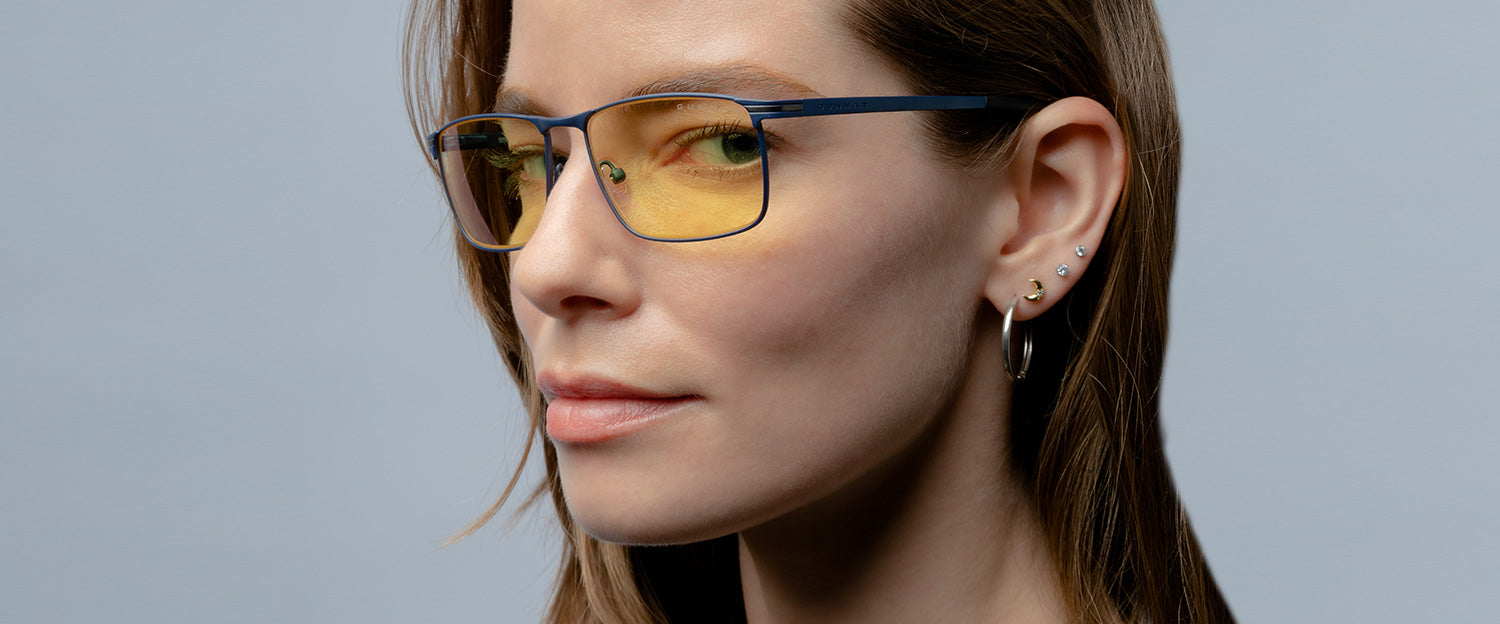In this detailed photograph, we see a young woman of Caucasian descent, appearing to be in her late 20s to early 30s, highlighted against a plain medium gray background. The image captures her from the neck up, with the top part of her head slightly cropped out. Her long, straight brown hair is tucked behind her ears, showcasing her array of ear piercings. She has a total of four piercings: two single stone studs, a small gold crescent moon stud, and a silver hoop earring. Her thin-rimmed glasses, which are navy blue, feature light yellow-tinted lenses that give a slight yellow hue to the whites of her eyes. She wears a hint of pink chapstick and exhibits a confident, slightly serious expression, with her head turned slightly to the left and her eyes engaging directly with the viewer.